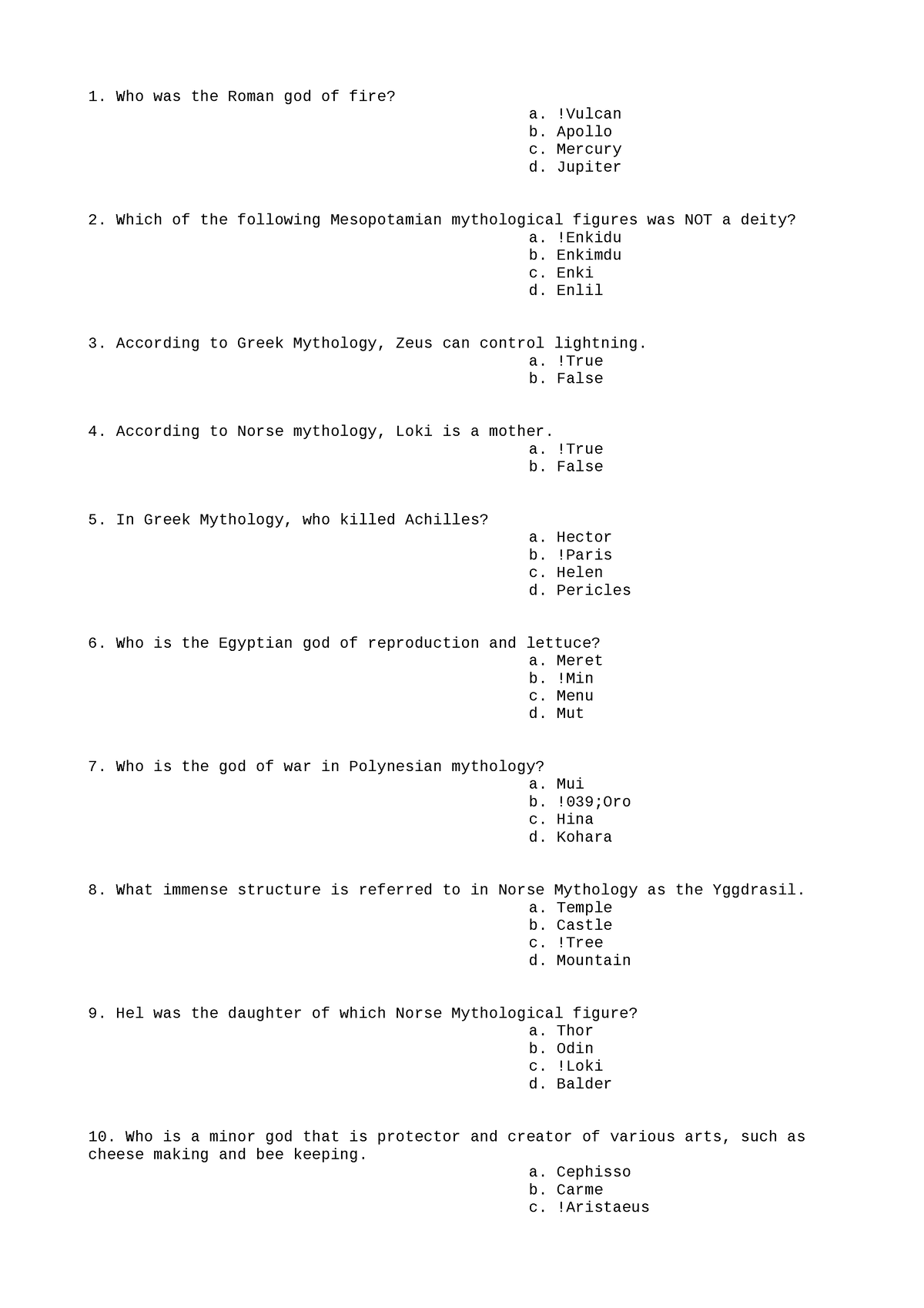The image features a white background with a series of questions and answers, although it is somewhat blurry due to zooming in, making the text difficult to read. Here's a detailed breakdown of the visible questions:

1. Who was the Roman God of fire?
   - A) Vulcan
   - B) Apollo
   - C) Mercury
   - D) Jupiter

2. Which of the following Mesopotamian mythological figures was not a deity?
   - A) Enkidu
   - B) [Illegible]
   - C) [Illegible]

3. According to Greek mythology, Zeus can control lightning.
   - A) True
   - B) False

4. According to Norse mythology, Loki is a mother.
   - A) True
   - B) False

5. In Greek mythology, who killed Achilles?
   - A) Hector
   - B) Paris
   - C) Helen
   - D) Pericles

6. Who is the Egyptian God of reproduction and lettuce?
   - [Illegible]

7. Who is the God of war in Polynesian mythology?
   - [Illegible] 

The questions span various mythologies, including Roman, Mesopotamian, Greek, Norse, Egyptian, and Polynesian. The image provides multiple-choice answers for most questions, though some text remains unclear due to the image's blurriness.